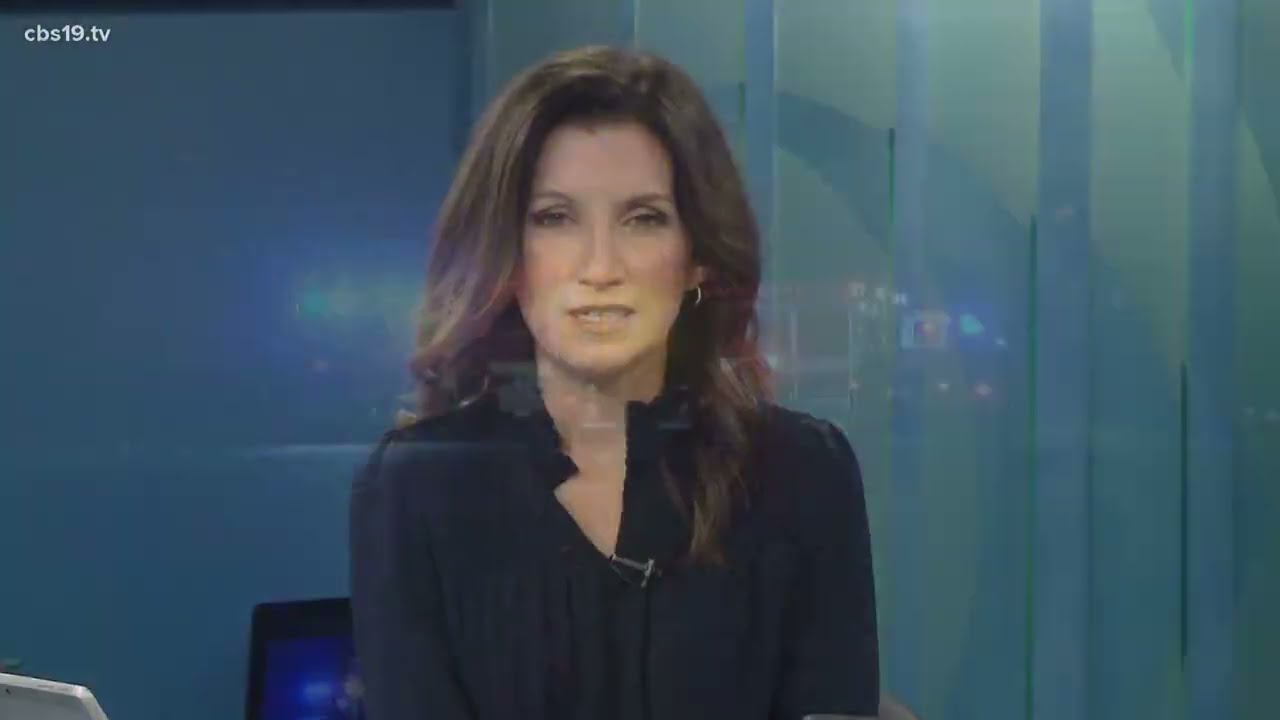The image features a female newscaster with long, flowing brown hair parted to the right and extending past her shoulders. She is dressed in a black long-sleeved top with a V-neck and ruffly collar, accessorized with small hoop earrings and a lapel microphone clipped to her shirt. She has a serious expression, with her mouth forming a straight line. The background is a mix of blue and greenish-blue hues with vertical striping. In the upper left corner, the text "cbs19.tv" is visible. A laptop with a silver finish is positioned in front of her, partially visible in the bottom left corner, along with a computer monitor behind her. Additionally, remnants of a previous news story involving a fire truck are faintly superimposed on the screen behind her, indicating that the image was captured during a transition of segments in a newscast. The photo is horizontal and rectangular in orientation.